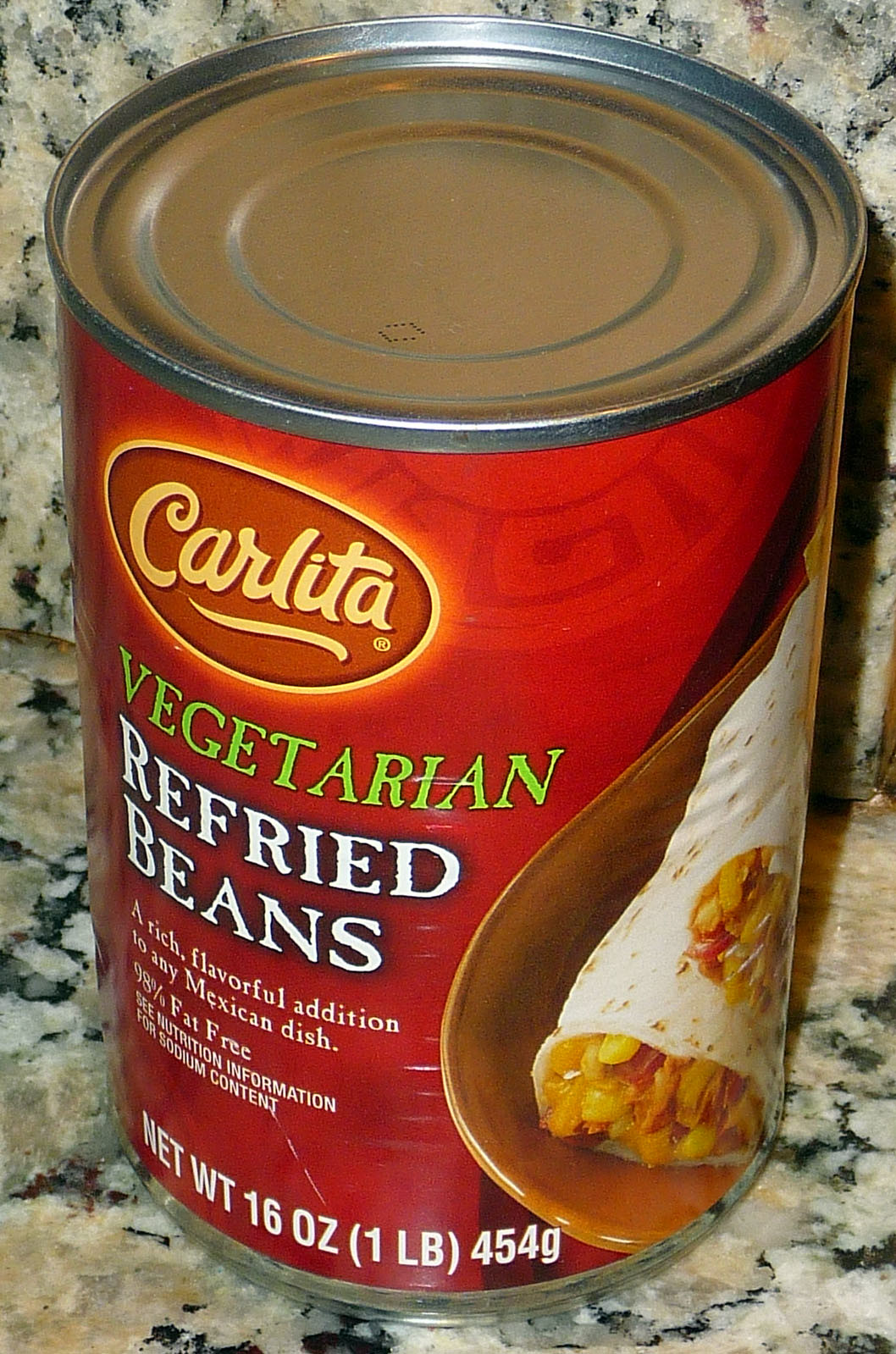The photograph depicts a close-up view of a 16-ounce can of Carlita brand refried beans, prominently displayed on a granite countertop with a tan, white, and black pattern. The can features a metal top with a dark gray ring around its edge. The label is predominantly red, with an oval-shaped logo at the top that reads "Carlita" in yellow script on a darker rust-colored background. Below this, "vegetarian" is written in bright green letters, followed by "refried beans" in bold white letters outlined in black. An additional tagline describes the beans as "a rich flavorful addition to any Mexican dish," alongside a declaration of being "100% fat-free." The can's net weight of 16 ounces (1 pound, 456 grams) is clearly noted at the bottom. To the right on the label, there is an illustration of an enchilada filled with refried beans, set on a brown plate.